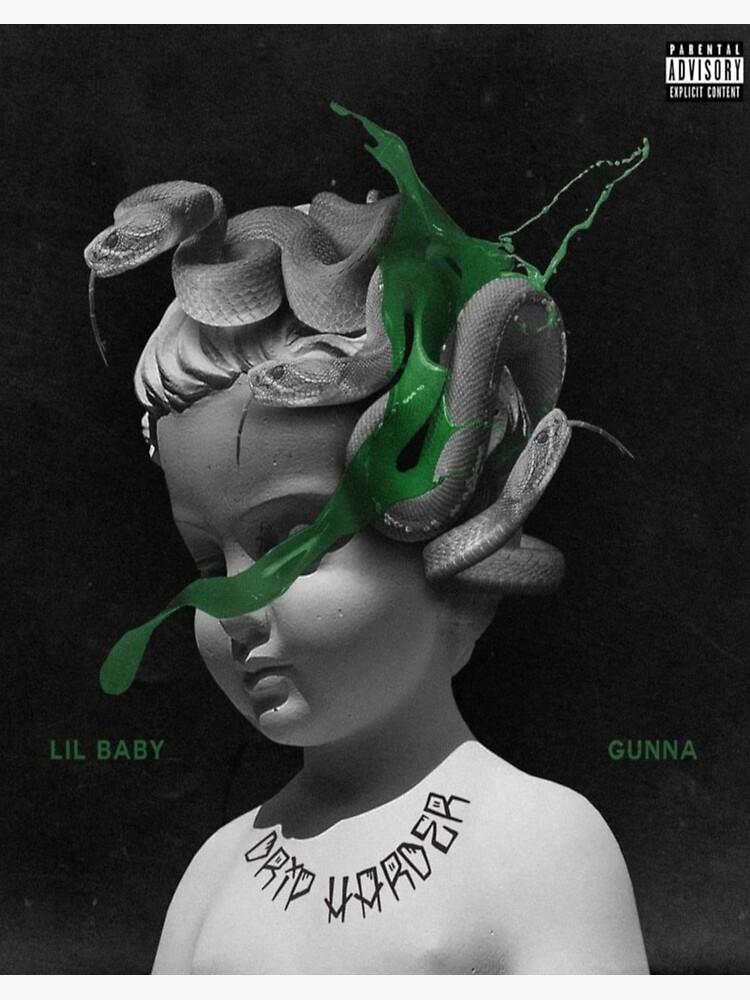The album cover features a 3D illustration with a black background. The central focus is a stone statue of a child, appearing around four years old, captured from the top of the head to mid-chest. The child’s head, adorned with three stone snakes, is facing slightly downward to the bottom left, eyes closed. Green paint splashes across the head and trails down the child's face, adding a dynamic contrast against the gray stone. Around the child's chest is etched circular text reading "Drip Harder." Flanking the statue, on the left side in green text, is "Lil Baby" and on the right in similar lettering is "Gunna." In the top right corner, white text displays "Parental Advisory Explicit Content." The detailed, textured style combines both 3D illustration and graphic design elements.